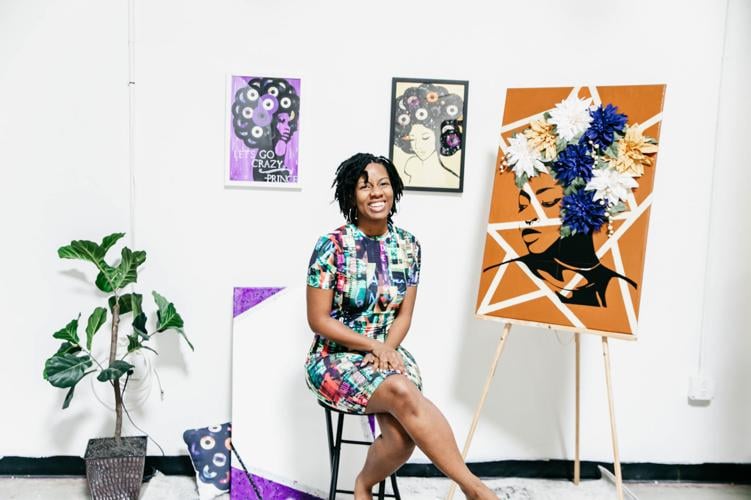This horizontally-oriented color photograph captures a bright, white-walled room with minimalistic black trim along the bottom. The floor is also white, contributing to the room's modern and clean aesthetic. The lighting showcases the various art pieces and the central figure in vivid detail.

Seated comfortably on a stool in the center of the room, a smiling African-American woman, possibly aged between 20 and 30, looks directly at the camera. Her right leg is crossed over her left, exuding a relaxed demeanor. Her medium-length black hair frames her face, and she wears a knee-length dress adorned with a vibrant, artistic checkered pattern in shades of red, orange, green, and other colors, reminiscent of a modernized madras style.

To her right stands an easel holding a striking mixed-media artwork featuring an African-American woman’s profile against an orange background. The woman in the painting has her hair represented by an array of blue, yellow, and white flowers, which appear to come off the canvas, enhancing the three-dimensional effect.

Behind the seated woman, two pieces of art are prominently displayed on the wall. The left painting has a vivid purple background with an African-American woman whose large hair is stylized to look like vinyl records. There's a notable title on this piece: "Let’s Go Crazy Prince." The right painting mirrors this style with a white background and also features a woman with record albums forming her hair.

Additionally, directly behind the woman is a large blank canvas leaning against the wall, hinting at potential future art, with a hint of purple, possibly part of an easel. To the far left of the photograph stands an indoor plant with wide leafy greens, adding a touch of nature, potted in a robust brown wooden vase. Further details include a light switch and two white-painted pipes extending vertically along the wall's right and left sides, completing the composition of this multifaceted and artistic room.